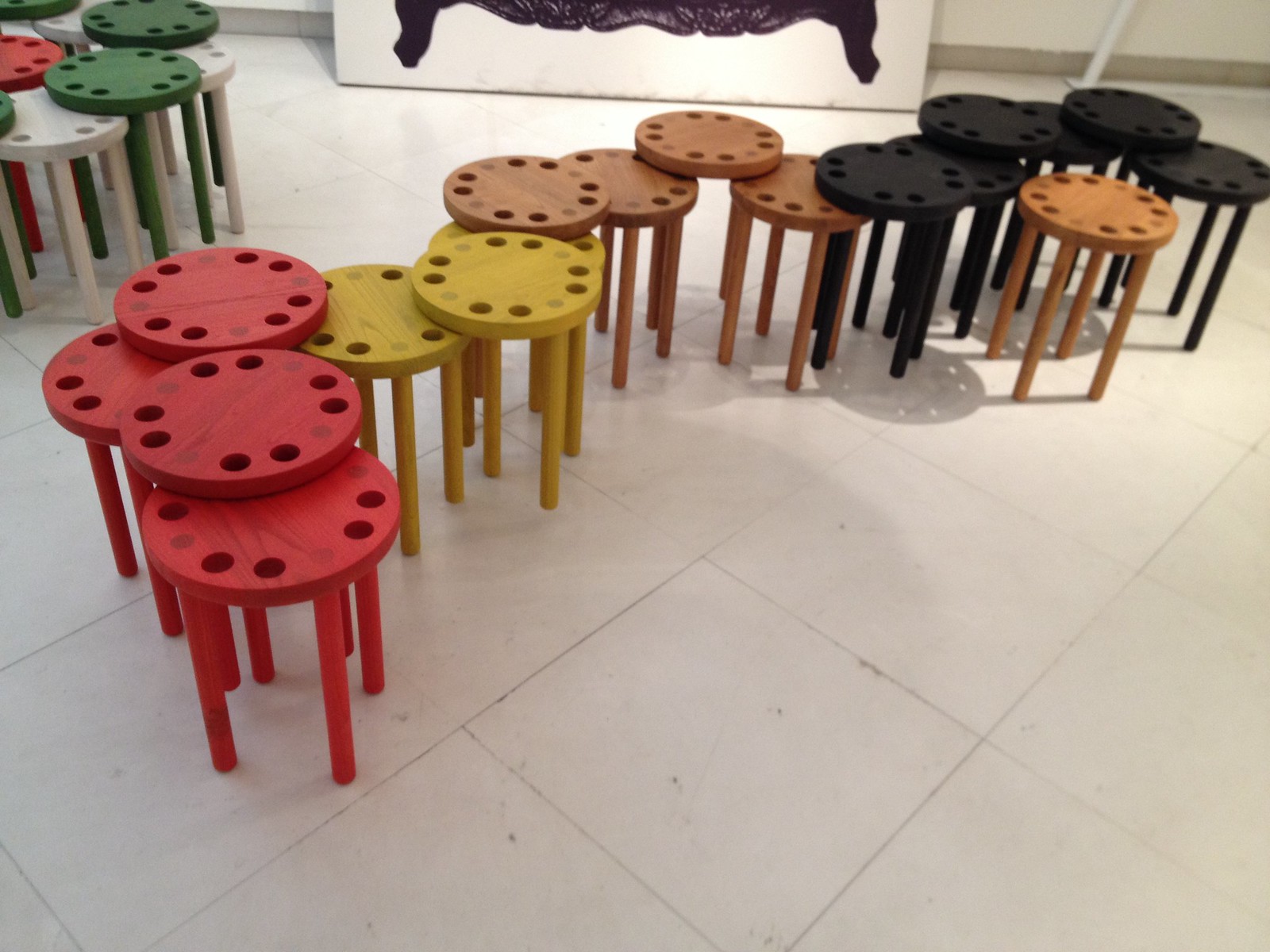The image shows a variety of interlocked stools arranged in a stacked, zigzagging pattern on a white tiled floor with diamond-shaped tiles. Each stool has four legs and a round top with a rotary dial-like design featuring holes in corresponding colors. Starting from the left, there are red, yellow, natural wood brown, black, green, and white stools, arranged in varying heights as if forming stepping stones. The stools' tops and holes share matching colors: red stools with red holes, yellow with yellow, and so on. In the background, there is a white wall with gray trim and a painting or whiteboard with black elements. The stools vary in height, with some able to slide under others, adding depth and complexity to the arrangement. The predominantly playful and colorful setup is accentuated by the multi-colored pattern of the stools, creating a visually engaging scene.